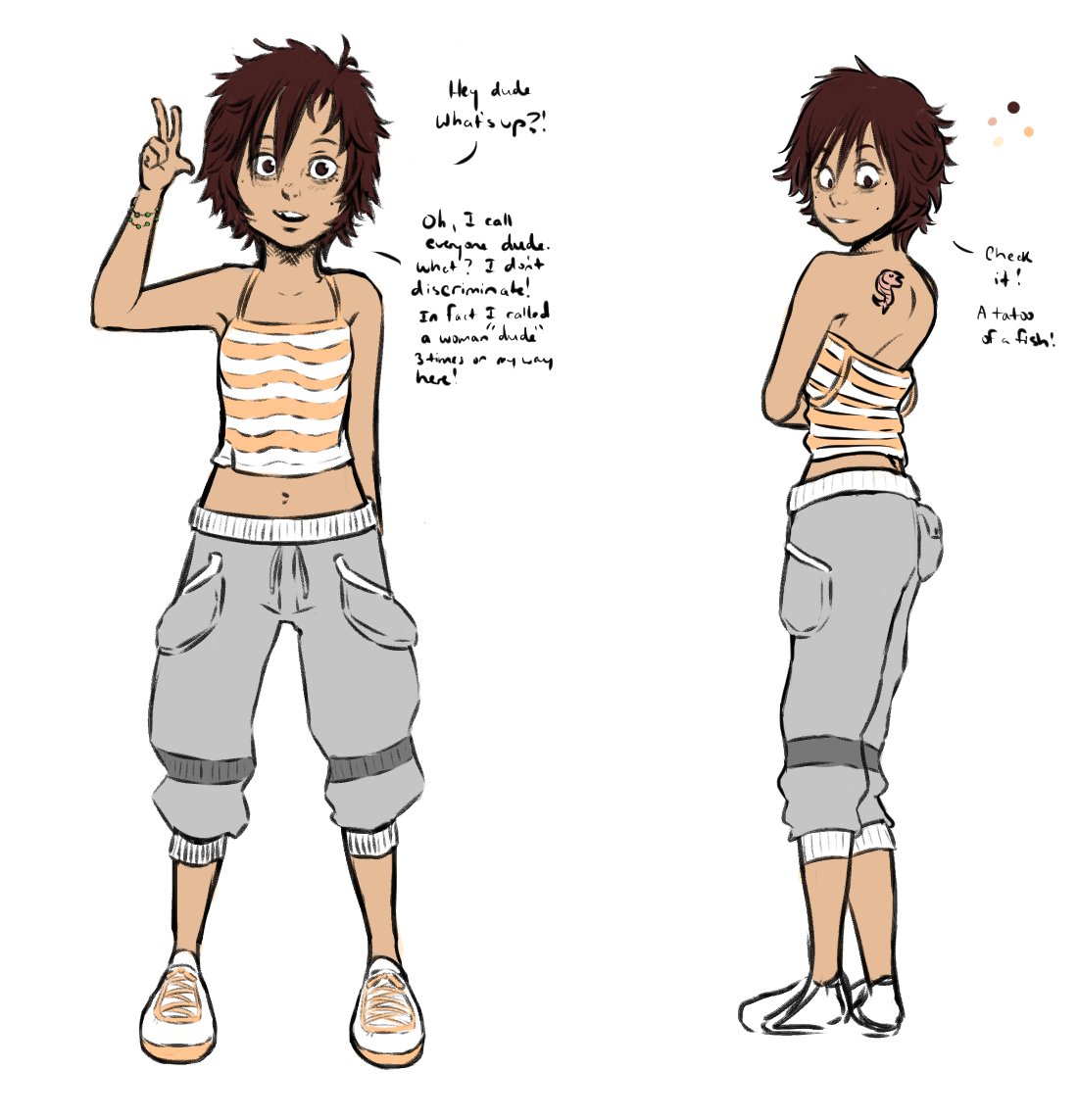This is a detailed drawing of the same cartoon woman shown in two different views: front and side. She has spiky brown hair and large brown eyes, exuding a friendly demeanor. In the front view, she wears a light orange and white striped halter top, revealing her midriff, paired with gray crop pants that sit low below her navel and are detailed with pockets and a ribbed band just below the knee. Her outfit is completed with white sneakers featuring orange laces. She is shown raising her right hand with two fingers extended.

The drawing features several pieces of text. In the first view, the woman says, "Hey dude, what's up?" and continues, "Oh, I call everyone dude, what? I don't discriminate. In fact, I called a woman dude three times on my way here."

In the second view, she is depicted from the side and slightly to her back, where a small sunfish tattoo is visible on her upper left shoulder. The text next to her reads, "Check it, a tattoo of a fish." Her spiky brown hair and overall attire add to her distinct, animated look, highlighted by her expressive dialogue and confident posture.